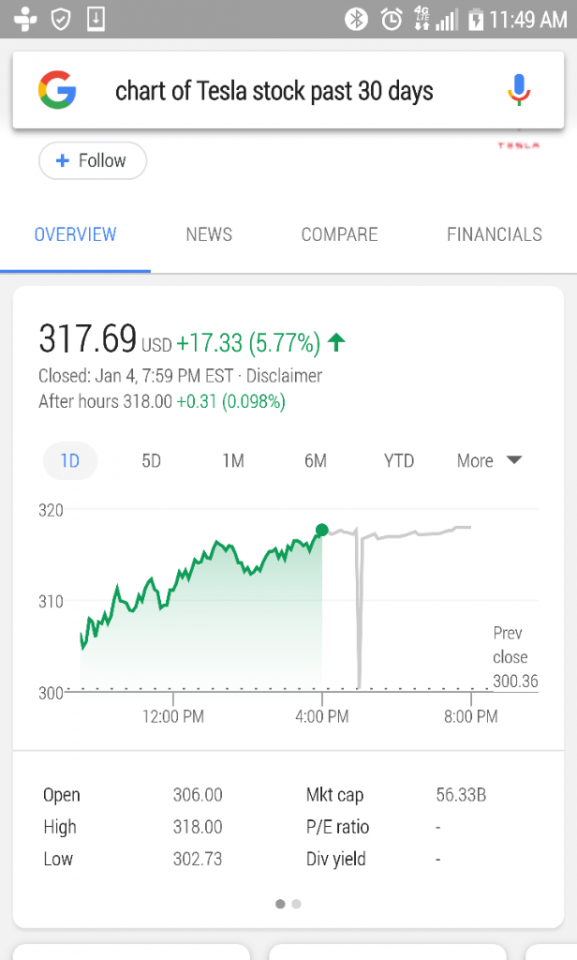The image depicts a smartphone screen captured at 11:49 AM, showing a mostly charged battery and available signal bars. At the top, there's a Google search bar. Below it, the display features a stock chart from the past 30 days, labeled with tabs such as 'Overview,' 'News,' 'Compare,' and 'Financials.'

Currently, the stock is valued at $317.69 USD, with an increase of $17.33 or 5.77% from the last close on January 4th at 7:59 PM Eastern Standard Time. A disclaimer notes that after-hours trading lists the stock at $318.00, a slight increase of $0.31 or 0.098%.

The chart illustrates varying stock values, displaying time markers at 12 PM, 4 PM, and 8 PM. The green line on the chart starts before 12 PM, roughly at 10 or 11 AM, at a value around $305. It shows a dip around noon but climbs up to approximately $310 later in the day.